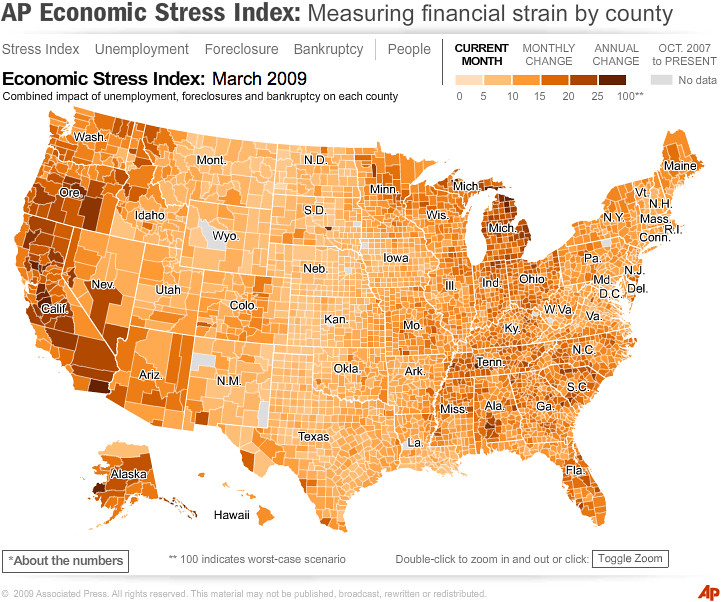This infographic, titled "AP Economic Stress Index: Measuring Financial Strain by County" for March 2009, presents a detailed map of the United States where each state or county is color-coded to reflect varying levels of economic stress. The legend indicates that lighter-colored areas represent lower stress, while darker-colored areas signify higher stress levels. The highest stress concentrations are seen on the West Coast and in Alaska, whereas the Midwest and some parts of the Northeast show the least stress, with the Southeast displaying mid-range stress levels. The index measures the combined impact of unemployment, foreclosures, and bankruptcy on each county. Additional information such as "About the Numbers" and an explanation that a score of 100 indicates the worst-case scenario is provided below the graph, along with instructions to use the Toggle Zoom button to explore the map further.